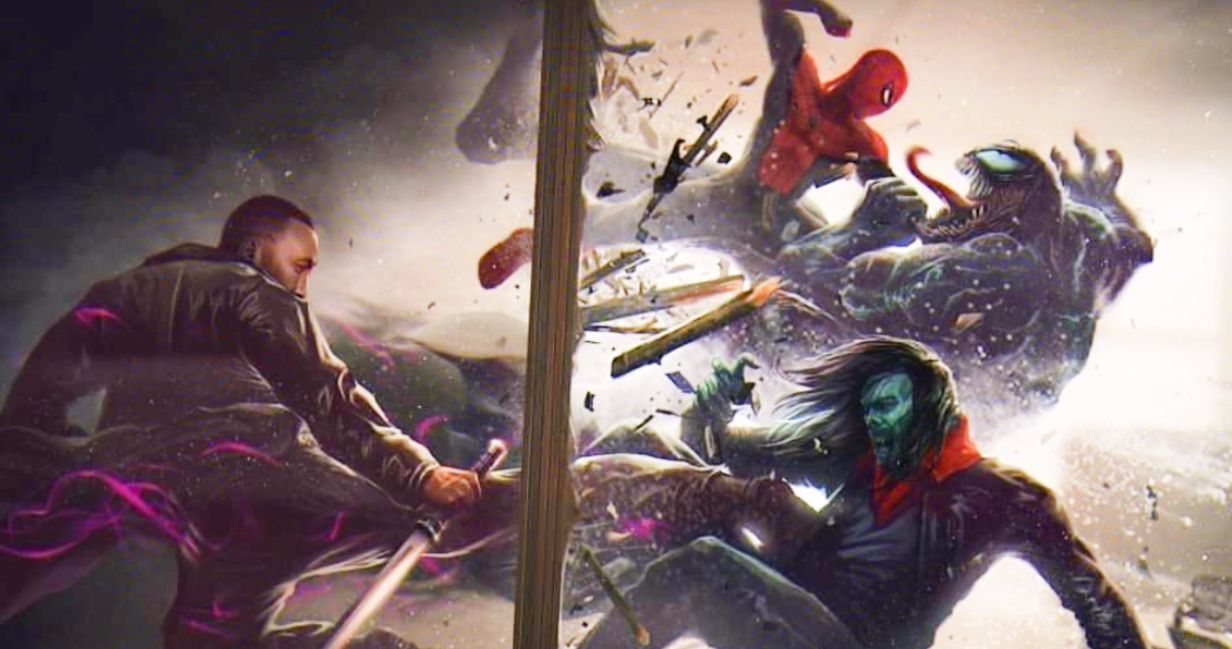The image is an intricate, animated illustration typical of a movie storyboard featuring a dynamic superhero battle. On the left-hand side, an African American man with a katana held upside down is attired in a black jacket with purple accents. He faces off against a villain with a bluish-green face, long black hair, a leather jacket, and a red cloth around his neck. The central area is dominated by a splintered tree, adding to the chaotic atmosphere. In the upper right, Spider-Man and Venom engage in a fierce, suspended punching match. Both duels are intense and appear to be occurring mid-air, emphasizing the action-packed scene.